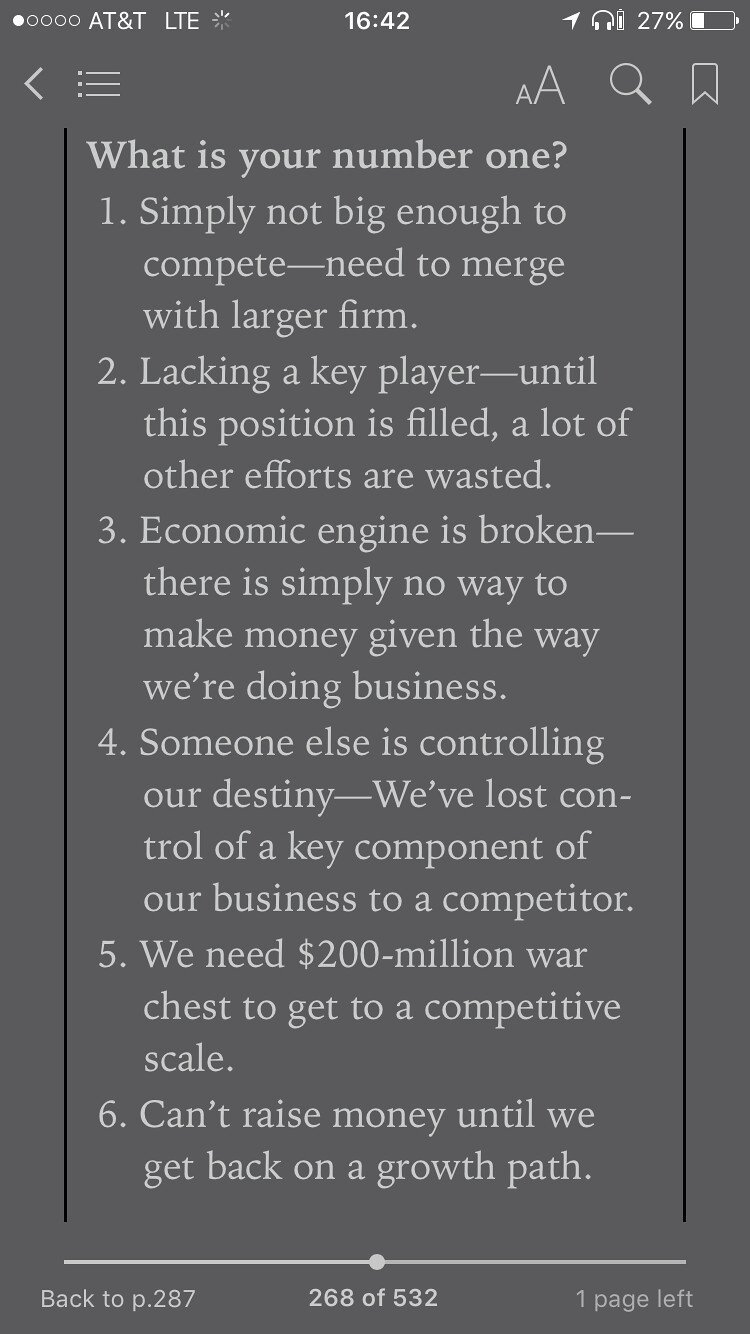The image is a tall rectangular screenshot taken from an iPhone displaying the AT&T LTE service, time 16:42, and a battery life of 27%. The background is dark gray with white text, resembling a note from a notes app. The note is titled in bold white letters "What is your number one?" and lists six issues faced by an organization. The listed issues are: 1. Simply not big enough to compete, suggesting the need to merge with a larger firm. 2. Lacking a key player, which wastes other efforts until the position is filled. 3. An economic engine that is broken, highlighting the inability to make money under the current business model. 4. Losing control of a key component of the business to a competitor. 5. Needing a $200 million war chest to achieve competitive scale. 6. Inability to raise money until a growth path is restored. The only colors used in the image are white and gray.